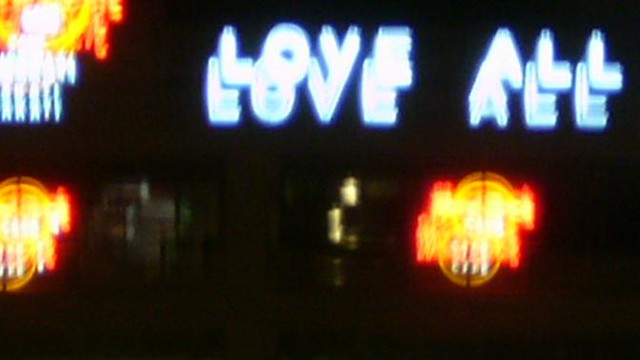The image is a horizontally aligned, landscape-oriented photograph, probably taken indoors at night due to its predominantly dark background. The main focus is on multiple neon signs with significant motion blur, indicating perhaps that the camera was shaking during the shot. At the top center-right, a blue or white neon statement reads "Love All," surrounded by a blue glow. This phrase appears twice, likely due to a motion blur effect. Below this, an orange neon Hard Rock Cafe logo is visible, featuring its signature circular design with some writing that is difficult to discern. Another similar orange neon sign appears in the top left corner and two-thirds down on the left side, all of which are also blurred but maintain a consistent orange-yellow glow. The unclear and overlapping nature of the signs contributes to the overall blurriness and difficulty in reading the text accurately.